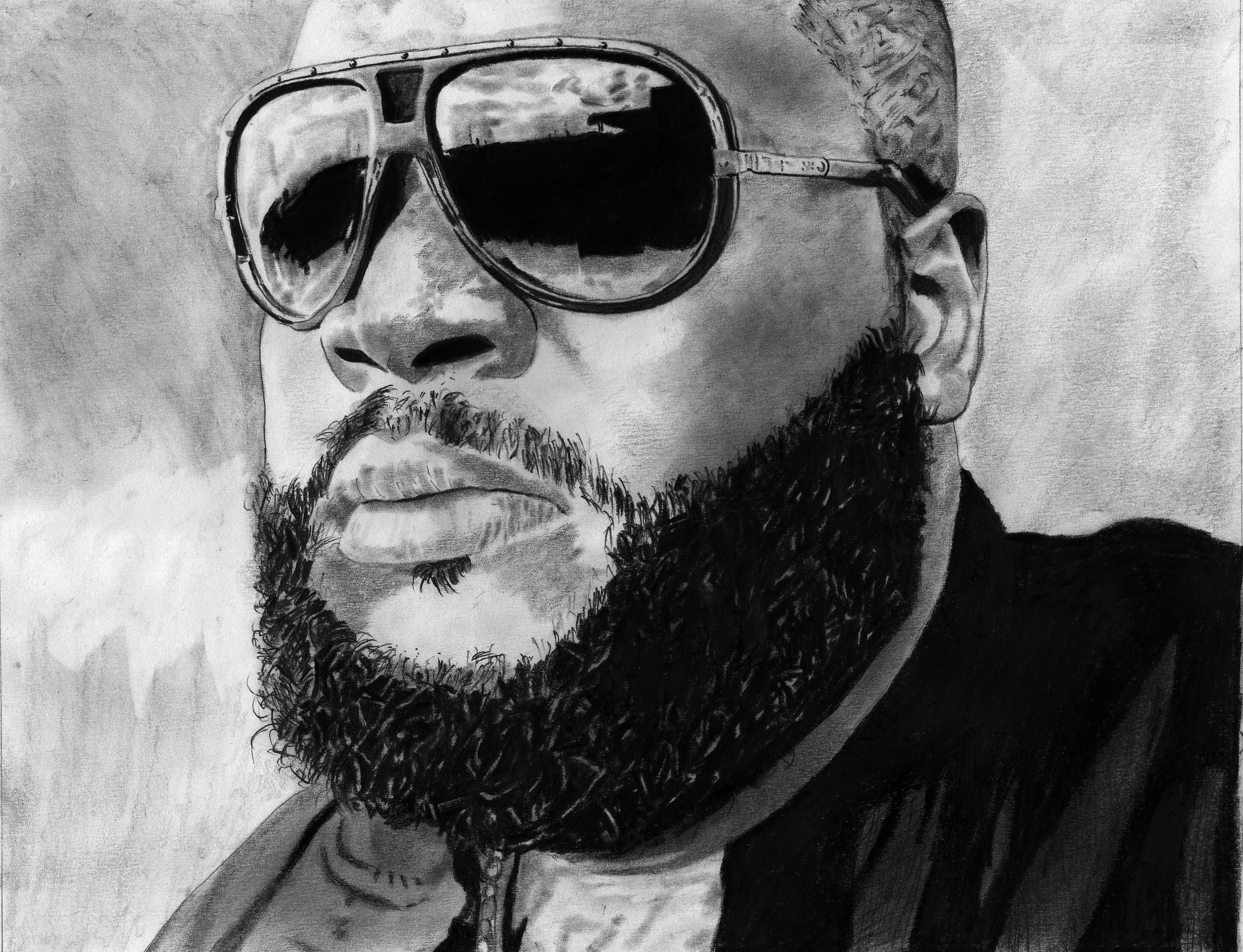The image is a detailed, black-and-white pencil drawing of rapper Killer Mike. The background is grayish, filled with pencil shading, giving it a textured look. Killer Mike is prominently featured, slightly off-center, with his gaze directed towards his right. He has a closely cropped shaved head, and his facial hair includes a thick, fuller beard and a thinner mustache. He is wearing dark sunglasses that reflect what appears to be an abstract cityscape. His attire consists of a black jacket worn over a grayish or white t-shirt, and he also has a chain around his neck. The drawing uses a range of tones from black to various shades of gray to create depth and detail. Overall, the image captures a serious and contemplative expression on his face.